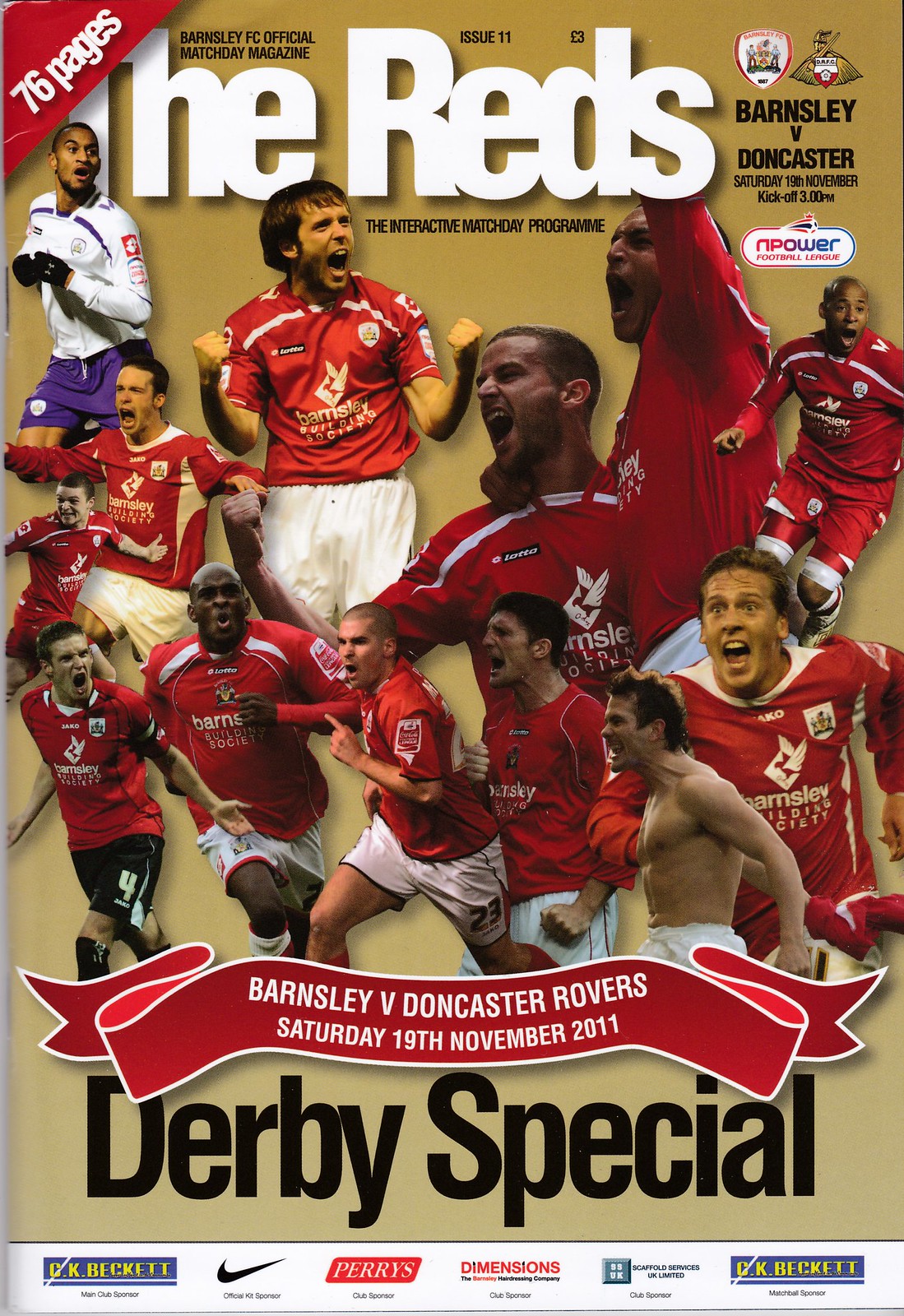The cover of this magazine, titled "The Reds," prominently features dynamic action shots of a soccer team, likely an homage to their dynamic spirit. The center of the cover is filled with players in various celebratory poses—fist-pumping, jubilant shouting, arms raised, and even one player with his shirt off. Most are clad in red jerseys with white shorts, except for a distinctive player in a white shirt and purple shorts, unmistakably the goalkeeper. The team's jerseys bear a prominent logo and the name "Beresley" just below the chest.

In the top left corner of the cover, a red triangle with white bold text states "76 pages," emphasizing the magazine's content. Adjacent to this, in large white letters, is the title "The Reds." Beneath this, the matchup "Barnsley vs. Doncaster" is highlighted, setting the theme for the issue. Further black text indicates the date and specifics: "Saturday, 19th November 2011, kickoff 3pm."

A red ribbon banner stretches across the lower part of the cover, repeating the matchup details and date, but in a more prominent and festive manner. Below this, in bold black letters, is the designation "Derby Special," indicating the significance of this particular game. The bottom edge of the cover is lined with advertisements, including recognizable logos like Nike, underlining the commercial support for the event. This cover combines vibrant visuals and detailed text to capture the excitement surrounding the Barnsley versus Doncaster Rovers derby on November 19, 2011.